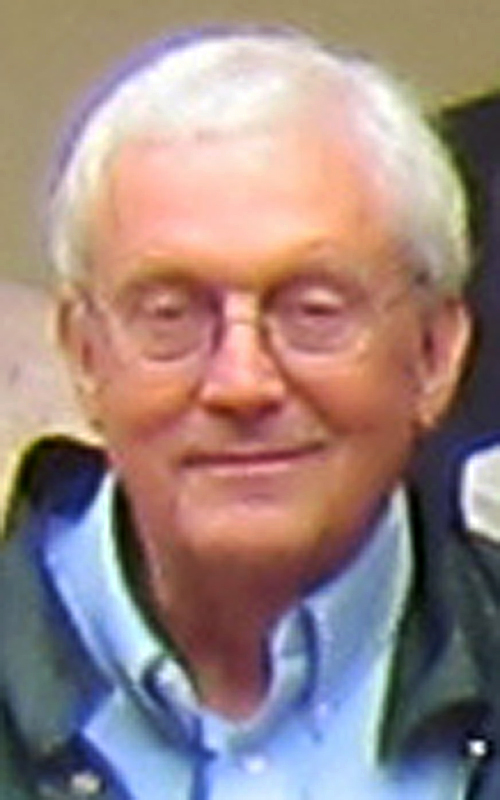This close-up headshot captures an elderly man indoors, possibly near a window judging by the faint hints of brown and black in the indeterminate background. The man has a round head with short white hair and appears to be slightly balding. His face is framed by rimless, roundish glasses that complement his gentle, closed-mouthed smile, which could be seen as a smirk. He is dressed in a blue button-down shirt with a black-trimmed collar visible underneath a suit jacket. The photograph, somewhat blurry, focuses tightly on his face, making it difficult to discern more specific details about the surroundings.